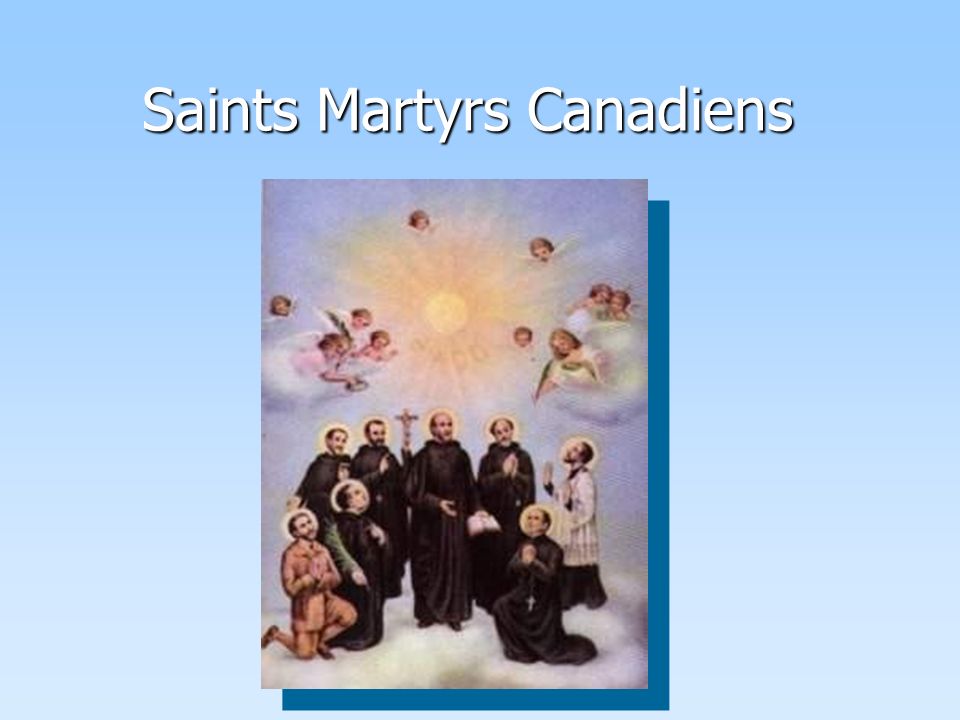This image, presented as an educational slide, features a religious scene within a horizontal rectangle that is slightly wider than it is tall. The background exhibits a smooth gradient from very light blue to an even lighter blue. At the top center, in white font with a black drop shadow, is the header text "Saints, Martyrs, Canadians," with the first letter of each word capitalized.

The central focus of the slide is a vertically oriented illustration, slightly off-center to the left, depicting a group of saints and monks enveloped in clouds. The saints, adorned in black cloaks, are both standing and kneeling, with halos around their heads, indicating their sanctity. Among them, one figure on the left edge is not wearing a brown robe and another on the right edge shares this distinction. Notable details include one saint wearing a white vestment over his black robe, another holding a crucifix aloft, and a third clutching a book in his left hand.

Above these figures, additional clouds harbor angels, cherubs, and young child angels, all contributing to the ethereal quality of the scene. A radiant sun illuminates the entire tableau from above, enhancing the divine atmosphere. The illustration itself is bordered by a dark blue rectangle, providing a subtle yet striking contrast against the lighter blue gradient of the background. The overall composition is slightly off-center, adding a unique visual dynamic to the image.